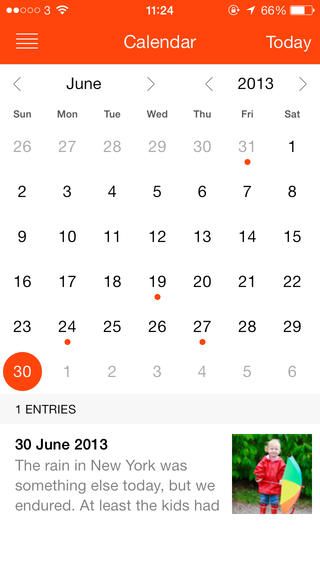A screenshot of a June 2013 calendar, taken from a mobile phone, features a striking orange bar at the top. The status bar indicates the device has 3G connectivity, Wi-Fi enabled, a 66% battery level, and is in airplane mode. The time is 11:24, and there is a lock icon as well as a context menu represented by four horizontal lines on the left side.

The calendar displays the current date—June 30th—highlighted with an orange circle and white text, while the dates from the previous and following months appear in gray. Below the calendar, there's an entry in bold indicating an event on June 30, 2013.

Accompanying the calendar is a charming image of a little girl dressed for the rain. She is adorned in a red raincoat, red galoshes, and blue rain pants, holding a multicolored umbrella to her right. She stands cheerfully in front of a bush, symbolizing the day's rainy weather in New York that was notably memorable, especially for the children.